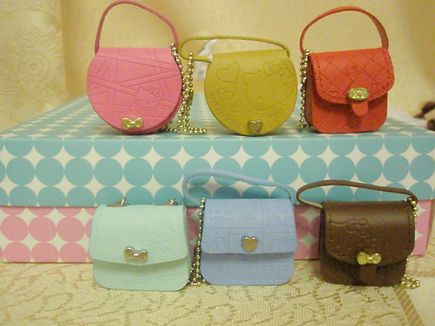This image showcases a set of six small handbags arranged in two rows, with three handbags in each row. The handbags on the top row sit atop a patterned rectangular box, with the top half featuring white and blue dots and the bottom half adorned with white and pink dots. These three handbags are colored pink, yellow, and red from left to right, each made from leather and featuring a single flap closure with either a heart or ribbon clasp. The handbag in pink prominently displays a Hello Kitty design etched on it, matching in style with the yellow and brown bags on the same row.

The bottom row of handbags is placed on a white rug with golden swirls. From left to right, the bottom row handbags are colored light mint, baby blue, and dark brown chocolate, each in a more rectangular shape. Notably, part of a Hello Kitty design can also be spotted on the light mint handbag on the left side. This cohesive and colorful arrangement highlights the playful yet elegant design of each handbag, set against a warm, light yellow background.